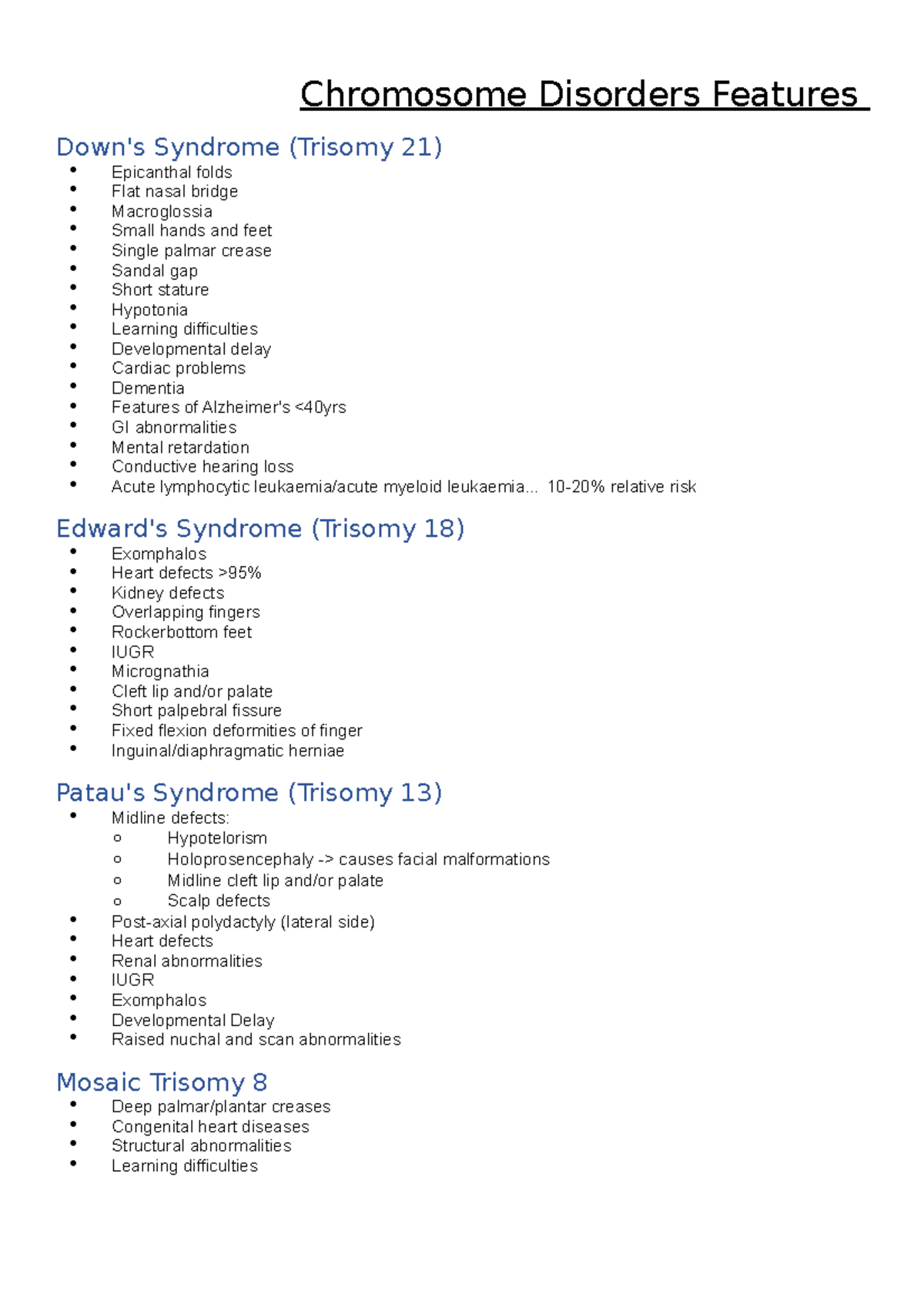Here is the cleaned-up and detailed descriptive caption for the image:

---

The background of the image is white. At the top center, in bold black text, it reads "Chromosome Disorders Features," with each word capitalized and underlined. The image is divided into multiple sections, each highlighting different chromosome disorders with corresponding features listed underneath.

1. **Down Syndrome (Trisomy 21)**
   - **Features:**
     - Epicanthal Folds
     - Flat Nasal Bridge
     - Macroglossia
     - Small Hands and Feet
     - Single Palmar Crease
     - Sandal Gap
     - Short Stature
     - Hypotonia
     - Learning Difficulties
     - Developmental Delay
     - Cardiac Problems
     - Early Onset Dementia (Features of Alzheimer's before 40 years old)
     - Gastrointestinal (GI) Abnormalities
     - Intellectual Disability
     - Conductive Hearing Loss
     - Increased Risk of Acute Lymphocytic Leukemia and Myeloid Leukemia (20% increased relative risk)

2. **Edwards Syndrome (Trisomy 18)**
   - **Features:**
     - Heart Defects (95% prevalence)
     - Kidney Defects
     - Overlapping Fingers
     - Rocker-Bottom Feet
     - Intrauterine Growth Restriction (IUGR)
     - Micrognathia
     - Cleft Lip and/or Palate
     - Short Palpebral Fissures
     - Fixed Flexion Deformities of Fingers

3. **Patau Syndrome (Trisomy 13)**
   - **Features:**
     - Midline Defects
     - Hypotelorism (decreased distance between the eyes)
     - Facial Malformations
     - Midline Cleft Lip and/or Palate
     - Scalp Defects

4. **Mosaic Trisomy 8**
   - **Features:**
     - Structural Abnormalities
     - Congenital Heart Diseases
     - Learning Difficulties

---